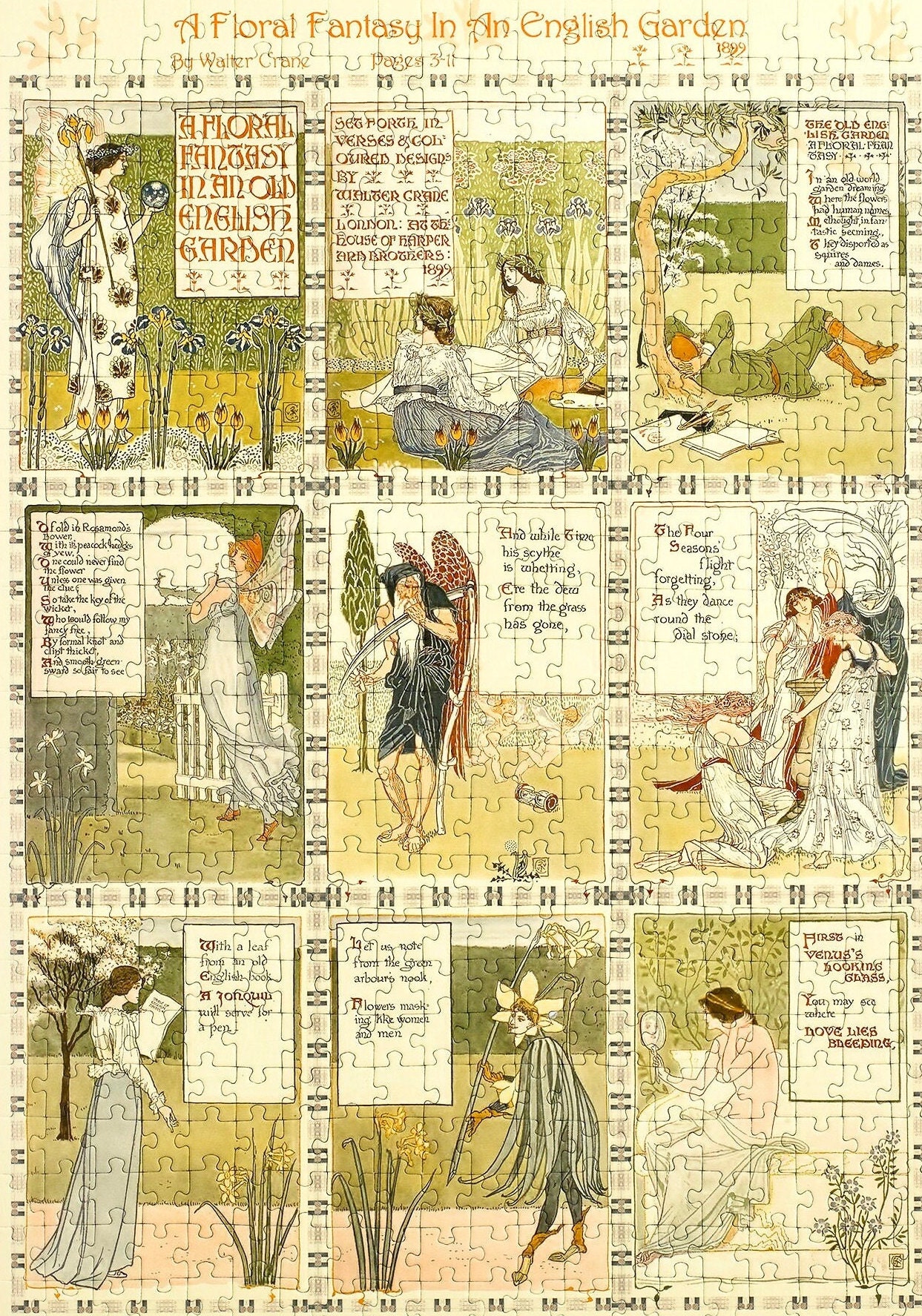The image depicts a complex, completed jigsaw puzzle with intricate details and a variety of scenes set against a pale yellow background. The puzzle is divided into nine interconnected blocks, each featuring a unique illustration and text, bordered by thin black outlines. The title at the top of the image, "A Floral Fantasy in an English Garden," is attributed to Walter Crane, set in a pale orange decorative font.

The top row consists of:
1. On the left, an angel holding a staff stands in a lush green garden.
2. In the center, two women are seated together against a green background.
3. On the right, a person is reclined against a brown tree branch, surrounded by green and yellow hues.

The middle row features:
1. On the left, a woman with long red hair beside some obscure writing.
2. In the center, a white-bearded man dressed in black.
3. On the right, three women, one kneeling, with another figure in the background.

The bottom row includes:
1. On the left, a woman reading a paper.
2. In the center, a woman with flower petals on her head, dressed in dark grey.
3. On the right, a woman in a pink shirt looking into a mirror, possibly seeing her reflection.

Each block includes text within white speech bubbles, though many of the words are difficult to decipher due to the decorative font. The scenes depict characters clad in vintage royal attire amidst a garden filled with flowers and trees, indicating storybook-like scenarios with various interactions and conversations taking place.